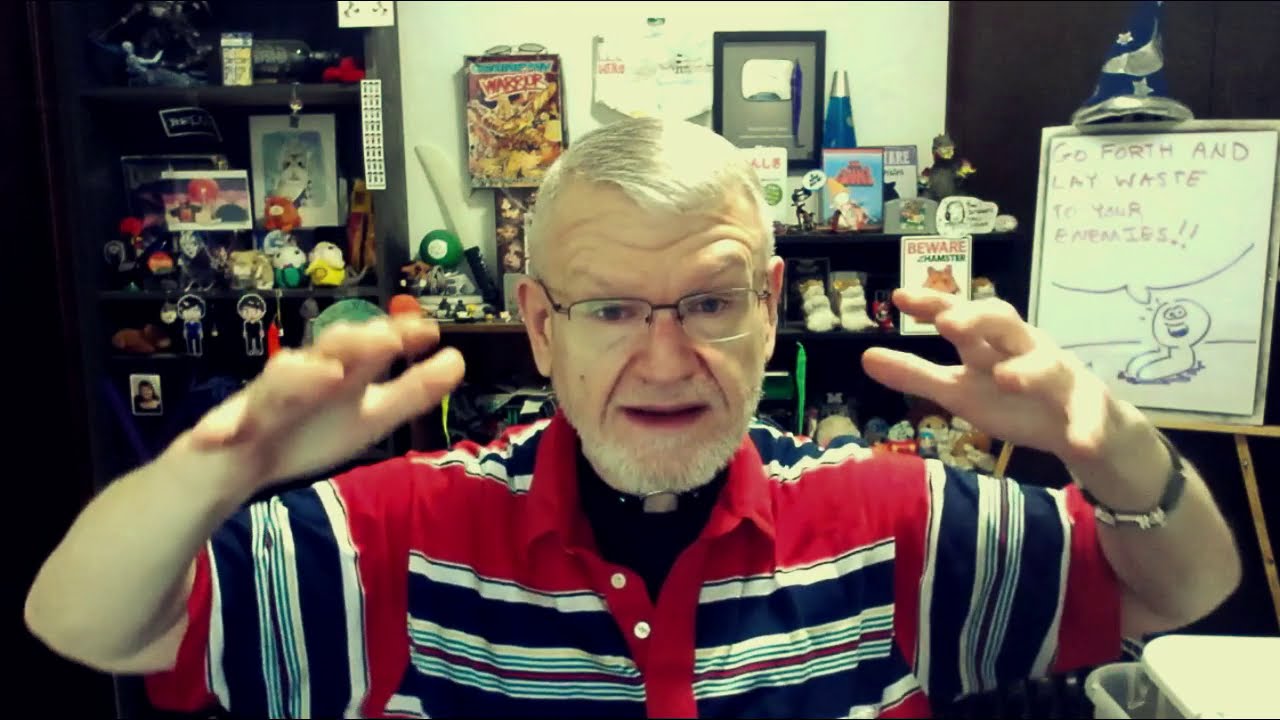In a vibrant and cluttered room filled with various collectibles, toys, and stuffed items, an older white gentleman stands center-frame in a horizontally rectangular, full-color photograph taken indoors. He has white hair, a white beard, and wears glasses. His attire includes a red short-sleeved button-down shirt with distinctive blue, light blue, and white horizontal stripes on the chest, shoulders, and arms, over what appears to be a black shirt, possibly complemented by a pastor’s collar. The man, who might be addressing the camera, holds his arms up dramatically, gesturing with his hands near his head. Behind him, a black shelf on a white wall is densely packed with assorted toys and bobbleheads. To his right, a whiteboard on an easel features a handwritten message, "Go forth and lay waste to your enemies," accompanied by a drawn cartoon character. Atop the easel sits a blue and silver wizard's hat, adding to the eclectic nature of the setting.